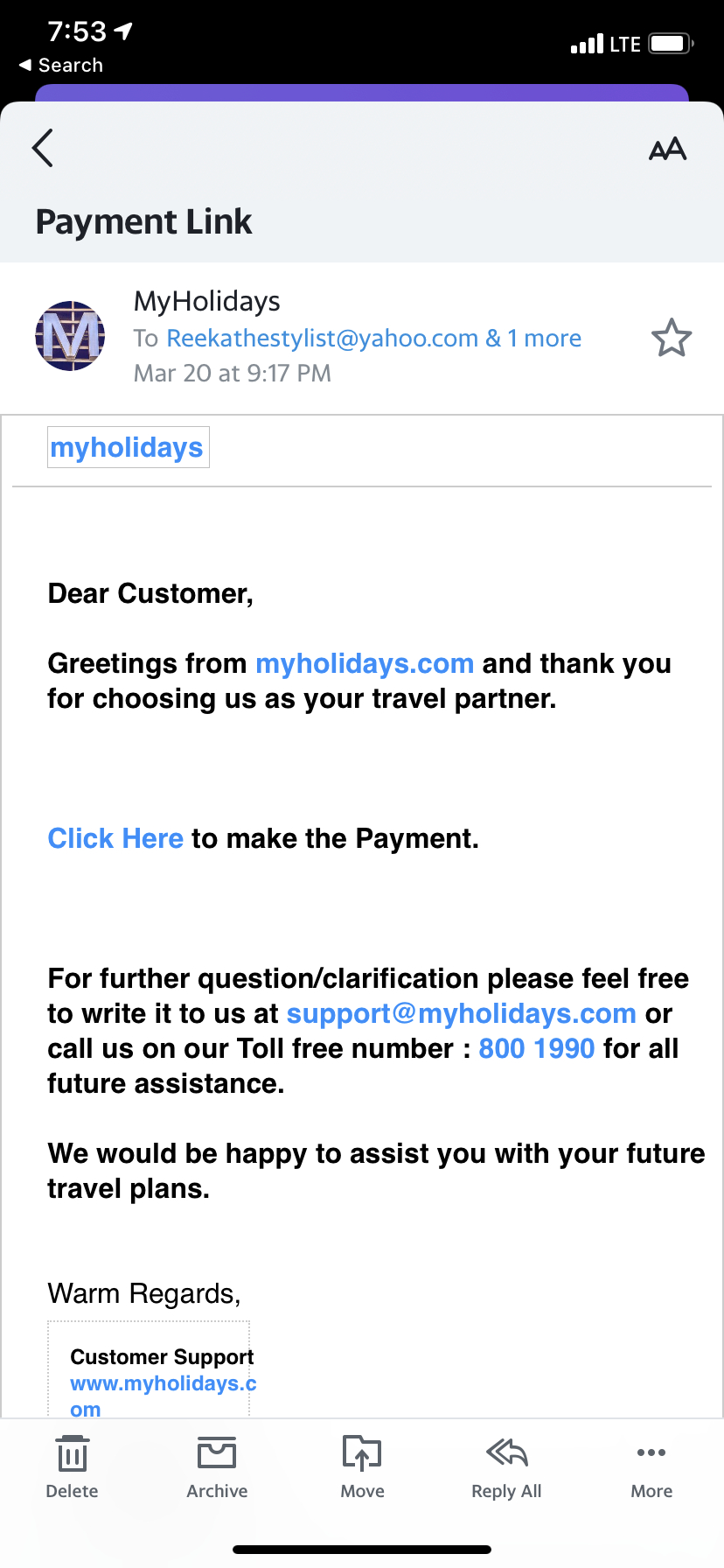A screenshot of a smartphone display shows the time as 7:53 with an arrow and search icon in the top left corner. The top right corner indicates full bars of LTE signal and an almost full battery. The screen displays the lower part of an email from My Holidays with the subject line "Payment Link." The sender's email address is listed as reekatestylist@yahoo.com, and the email was sent on March 20th at 9:17 p.m. The email header shows a star with two 'A's above it and a profile picture that features a white letter 'M' in front of window blinds.

The body of the email is highlighted with the phrase "My Holidays" in blue. It opens with: “Dear customer, greetings from myholidays.com and thank you for choosing us as your travel partner. Click here to make the payment. For further questions or clarification, please feel free to write to us at support@myholidays.com or call us on our toll-free number 800-1990 for all future assistance. We would be happy to assist you with your future travel plans. Warm regards, Customer Support, www.myholidays.com.”

Email management options such as "Delete," "Archive," "Move," "Reply All," and "More" are displayed at the bottom, with a faint black line running through the middle of these options.